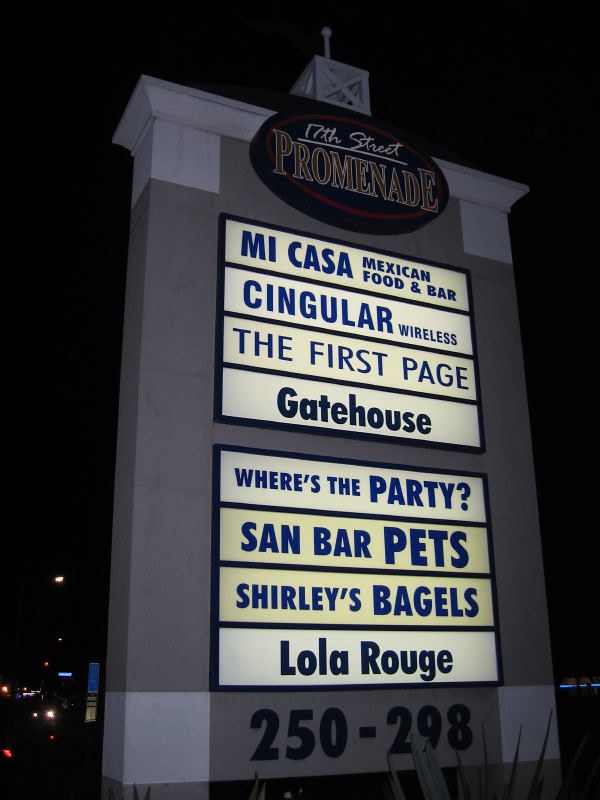A nighttime photograph captures a robust cement tower sign for a bustling shopping plaza, prominently displaying the name "17th Street Promenade" at the top. The signage includes various stores, all illuminated in blue font. The top slot advertises "Mi Casa Mexican Food and Bar," followed by "Singular Wireless," "The First Page," and "Gatehouse." After a brief space, additional businesses are listed: "Where's the Party," "Stand Bar Pets," "Shirley's Bagels," and finally "Lola Rouge" at the bottom. The sign also displays an address, "250-298," adding to the detailed navigation for visitors.